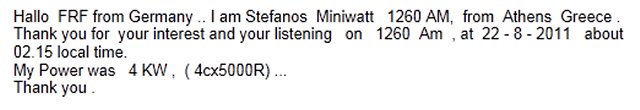The image consists of left-aligned black text on a white background, spread over five lines. The text reads: "Hello, FRF from Germany... I am Stephanos Miniwatt, 1260 AM, from Athens, Greece. Thank you for your interest and your listening on 1260 AM, at 22-8-2011, about 02:15 local time. My power was 4KW (4CX5000R)... Thank you." The text appears to be a QSL card, typically used to confirm a radio broadcast reception. This particular card confirms a transmission from Athens, Greece, picked up in Germany. The message is delivered in a straightforward, unadorned format with no additional graphics or borders.